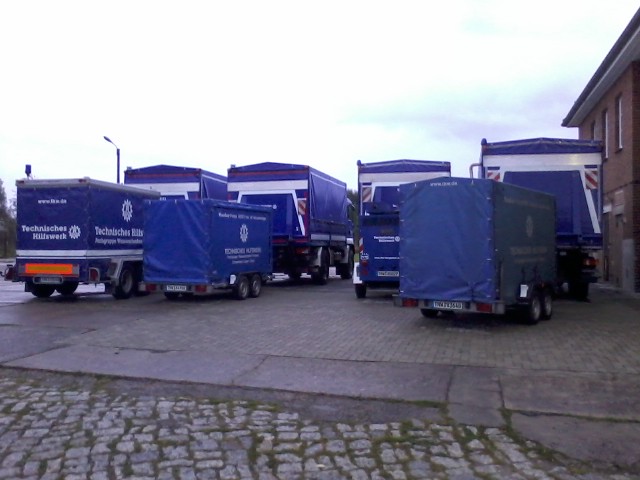In the photograph, four large industrial trucks with blue and white designs are prominently parked outdoors on a cobblestone-like cement surface. The trucks, three of which have matching blue and white trailers hitched behind them, offer a rugged industrial look, while the second truck from the right stands out as it lacks a trailer. The truck furthest to the right, along with the second from the left, has its trailer covered in blue plastic. Partially visible writing on the trucks, beginning with the letters "T-E-C-H", hints at a foreign language, though the exact message is indiscernible. 

The scene is set against a backdrop of a brown-brick building with a distinctive white and black roof, situated to the right of the parked trucks. Visible second-story windows suggest a business establishment. The sky above is a blend of fluffy white clouds with patches of blue visible, lending a serene, open-air atmosphere to the industrial setting.